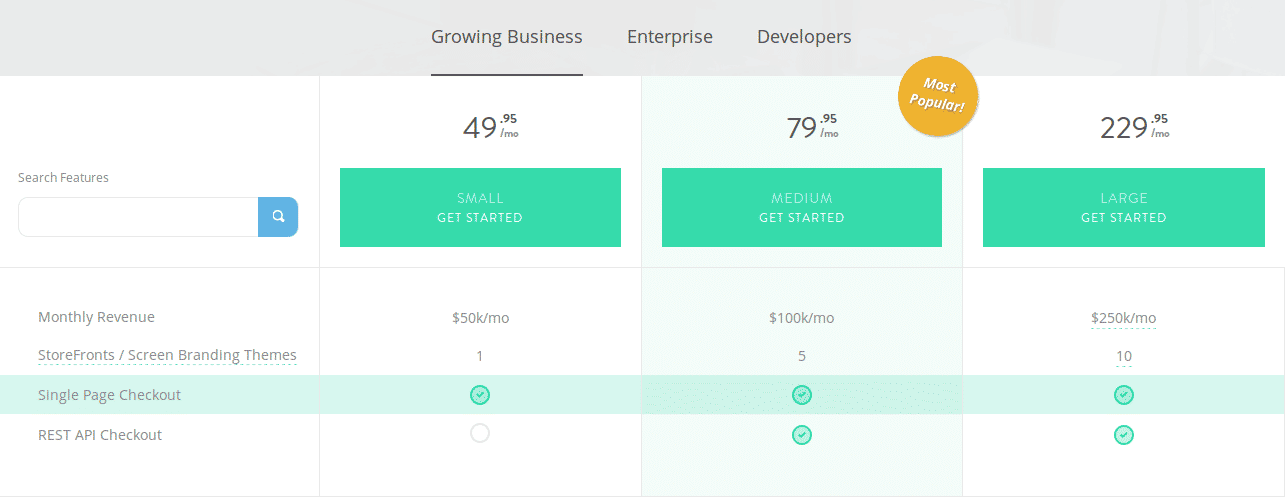This image displays a detailed pricing plan comparison for a growing business enterprise. The screenshot features four distinct columns under different sections: REST API Checkout, Single Page Checkout, and Storefront. Each section provides tiered options for Small, Medium, and Large businesses, highlighting the varying monthly revenues and corresponding packages.

- **Small Plan**: This plan, labeled "Get Started," offers a single page checkout option with a monthly revenue cap of $50K.
- **Medium Plan**: Highlighted with a translucent light green background and marked with a yellow circle indicating "Most Popular," this plan supports up to $100K in monthly revenue.
- **Large Plan**: Priced at $229 per month, this plan caters to businesses with revenues up to $250K per month.

Additionally, for enterprises and developers, there are specified sections allowing users to search and compare the features pertinent to their needs. This descriptive breakdown helps businesses choose the most suitable option according to their scale and requirements.